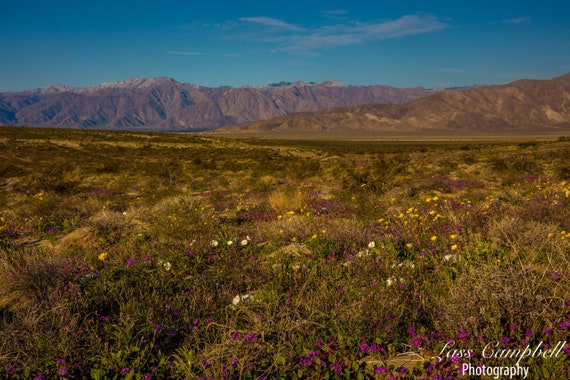This nature photograph captures a vast, desert-like valley, evoking the rugged beauty of a mesa landscape. The foreground is dominated by weedy, scrub brush vegetation, characterized by shades of brown and yellow, with sparse greenery. Scattered across the terrain are splashes of color from blooming flowers—vibrant yellows and subtle purples, marking the onset of a super bloom. The expansive scene is framed by a range of rocky mountains in the distance under a brilliant, clear blue sky, devoid of clouds. At the lower right corner of the image, a watermark reads "Last Campbell Photography" in a combination of cursive and plain white font, acknowledging the artist's work.